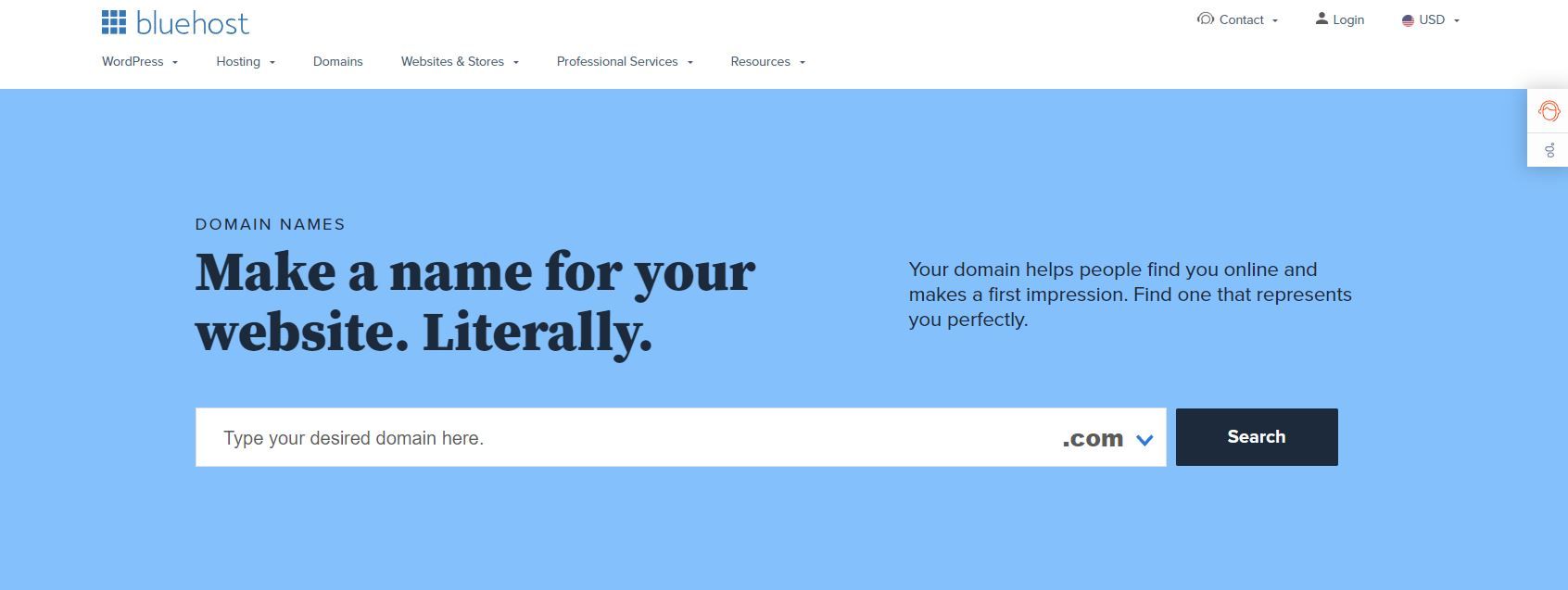This is a screenshot of the Bluehost webpage viewed on a desktop, tablet, smartphone, or laptop. At the top left corner, the Bluehost logo is prominently displayed, featuring the customary nine dark blue squares arranged to form a larger square. The company name "bluehost" is written next to the logo in lowercase letters with the text "B-L-U-E-H-O-S-T."

On the far right side of the header, there is a contact icon depicted as a thought bubble with a line, accompanied by a drop-down menu. Next to it, there is a silhouette of a person labeled "Login" and an American flag icon next to the text "USD," also with a drop-down menu for currency options.

Below the header, a navigation bar contains various tabs in black text, most with down arrows except for one. The tabs are labeled WordPress, Hosting, Domains (without a down arrow), Website and Stores, Professional Services, and Resources.

Beneath the navigation bar, a large blue section features a domain search interface. On the left side, the text "domain names" is displayed in black, while the bold black text reads "Make a name for your website." On the far right, the text "Your domain helps people find you online and makes a first impression. Find one that represents you perfectly" is written in thin black letters.

Centered in this section is a white search bar with the placeholder text "Type your desired domain here." To the right of the search bar, the text ".com" is displayed in bold black with a blue down arrow for selecting other domain extensions. Below the search bar, a dark blue button with the word "Search" written in white invites users to find available domains.

Finally, in the top right corner of the page, a small rectangle shows an egg icon inside a hexagonal red shape, coupled with a two-circle icon, symbolizing notifications or messages.